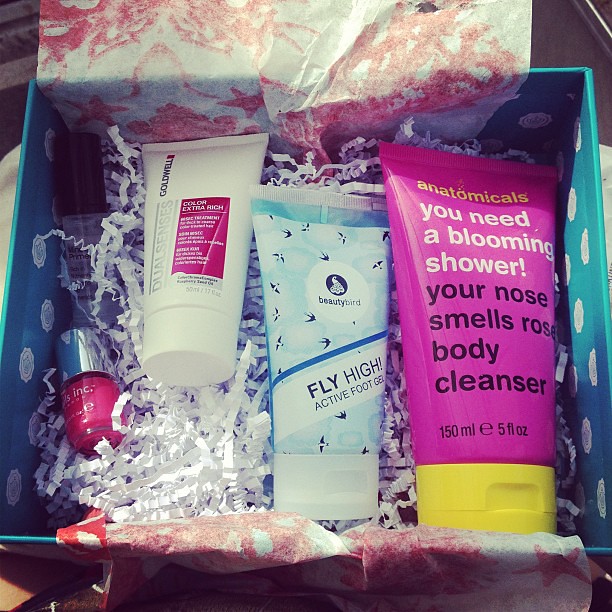This close-up color photograph showcases an open teal blue gift box adorned with white polka dots. Featuring white box stuffing and pink and white tissue paper spilling out, the box is filled with personal care and beauty products arranged neatly. Starting from the left, there's a small glass bottle of pink nail polish beside a clear nail polish bottle. Next to the nail polishes lies a white plastic tube of Dual Senses Goldwell Extra Rich Conditioning Gel. Adjacent to this, a blue and white plastic tube of Beauty Bird Fly High Active Foot Gel is positioned. Finally, the largest item in the box is a striking pink and yellow plastic tube labeled "anatomicals: you need a blooming shower, your nose smells rose body cleanser," which contains 150 milliliters or 5 ounces of product. This carefully curated selection of beauty essentials is nestled amidst decorative white confetti, making the entire presentation visually appealing and inviting.